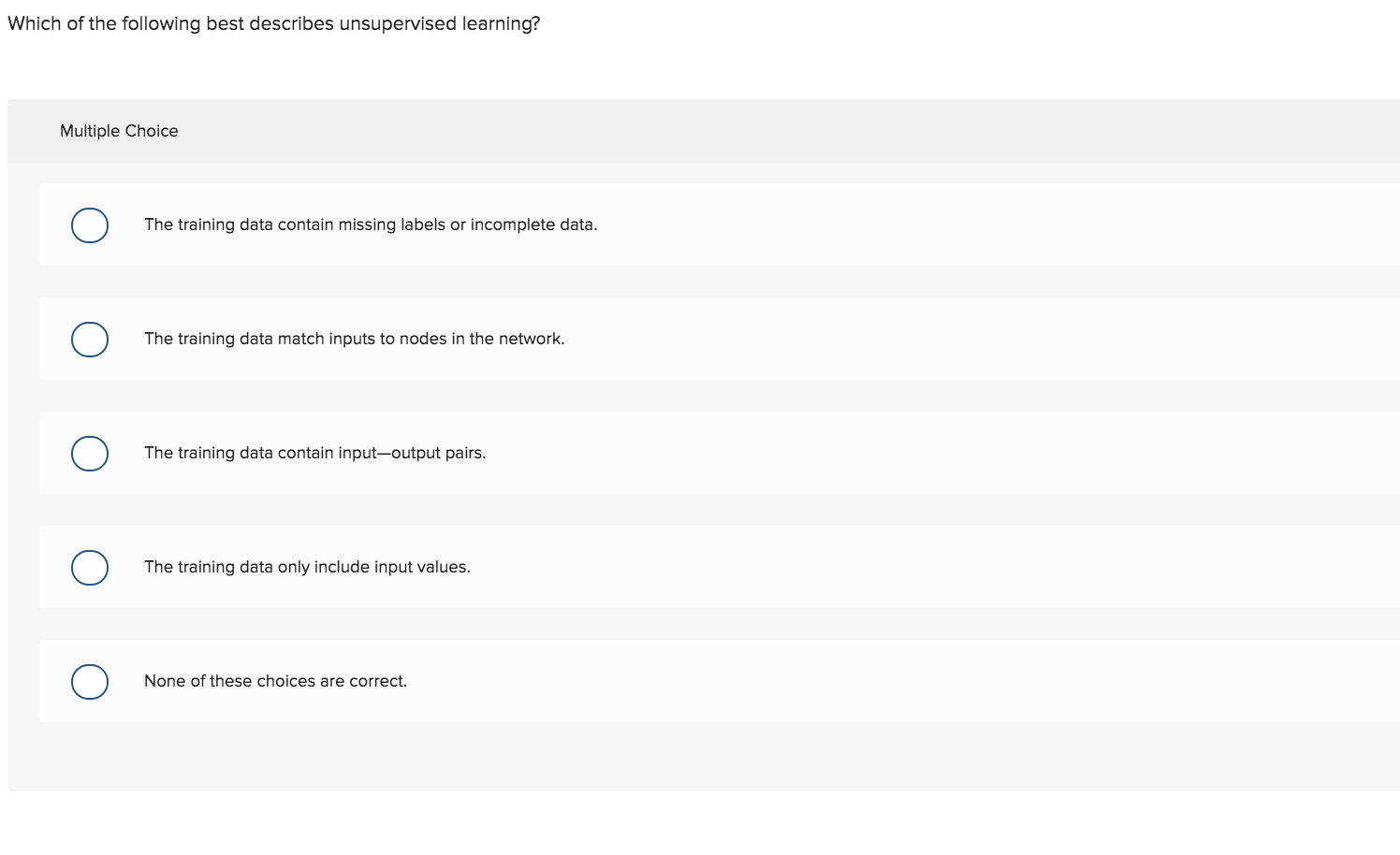This screenshot depicts a segment of an unidentified revision software or website designed to test the user's knowledge. The website lacks any visible logos but presents a question on a white background that reads: "Which of the following best describes unsupervised learning?" Below this, it is indicated that the question format is multiple choice. Five possible answers are listed:

1. The training data contains missing labels or incomplete data.
2. The training data matches inputs to nodes in the network.
3. The training data contains input-output pairs.
4. The training data only includes input values.
5. None of these choices are correct.

Each of these options is accompanied by a white circle with a blue outline, intended for selection. The absence of any ticks next to the circles suggests that the user has not yet selected an answer and may still be deciding which one is correct.